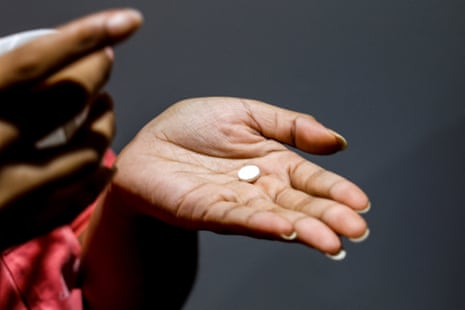The photograph features a close-up of a dark-skinned woman's hands against a dark gray background. Her right hand, positioned to the left of the image, is facing away from the viewer and partially obscures a container, although its label is not visible. Her left hand, which is centrally placed, has the palm upturned, showcasing a single white circular pill. The woman is wearing a red shirt that is visible in the lower left part of the image. The overall scene is brightly lit with natural light, which enhances the clarity and vividness of the colors in the photograph. The image does not include her face or any other text or numbers. The woman's long fingernails and the positioning of her hands strongly suggest she is presenting the pill to the camera.